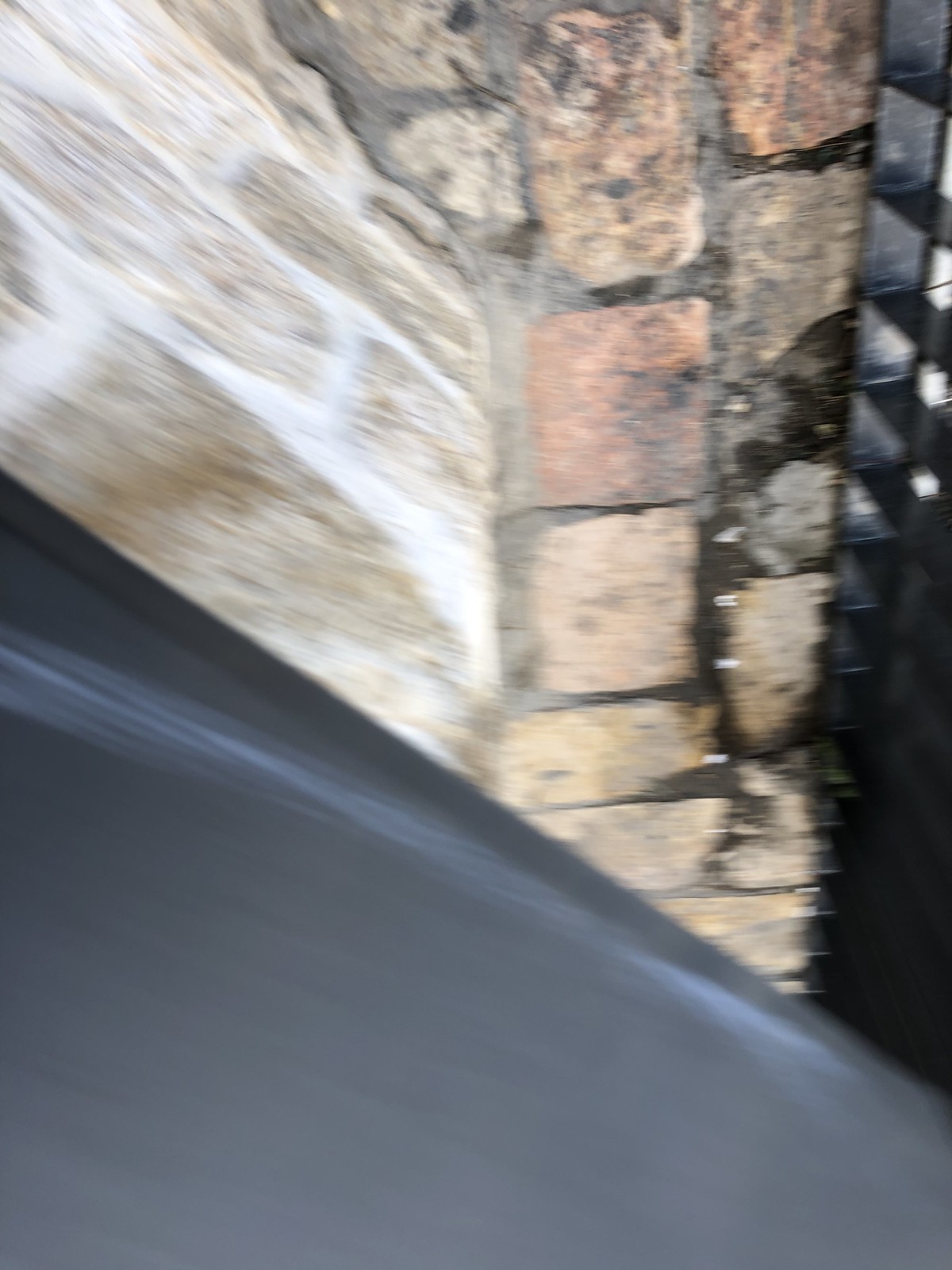This image presents a highly blurry scene, making it challenging to discern distinct elements. In the lower half to the bottom-left corner, a prominent black blob, possibly an object or shadow, occupies a significant portion of the frame. Directly above this dark area, a white line stretches horizontally, providing a contrasting boundary. Towards the upper section of the image, the scene transitions into a wall composed of bricks. On the left side, the bricks appear flat and aligned, while on the right side, the bricks are square-shaped and neatly stacked, showing more clarity compared to the rest of the picture. Despite the overall blurriness, these brick details are more distinguishable and offer a sense of structure within the image.